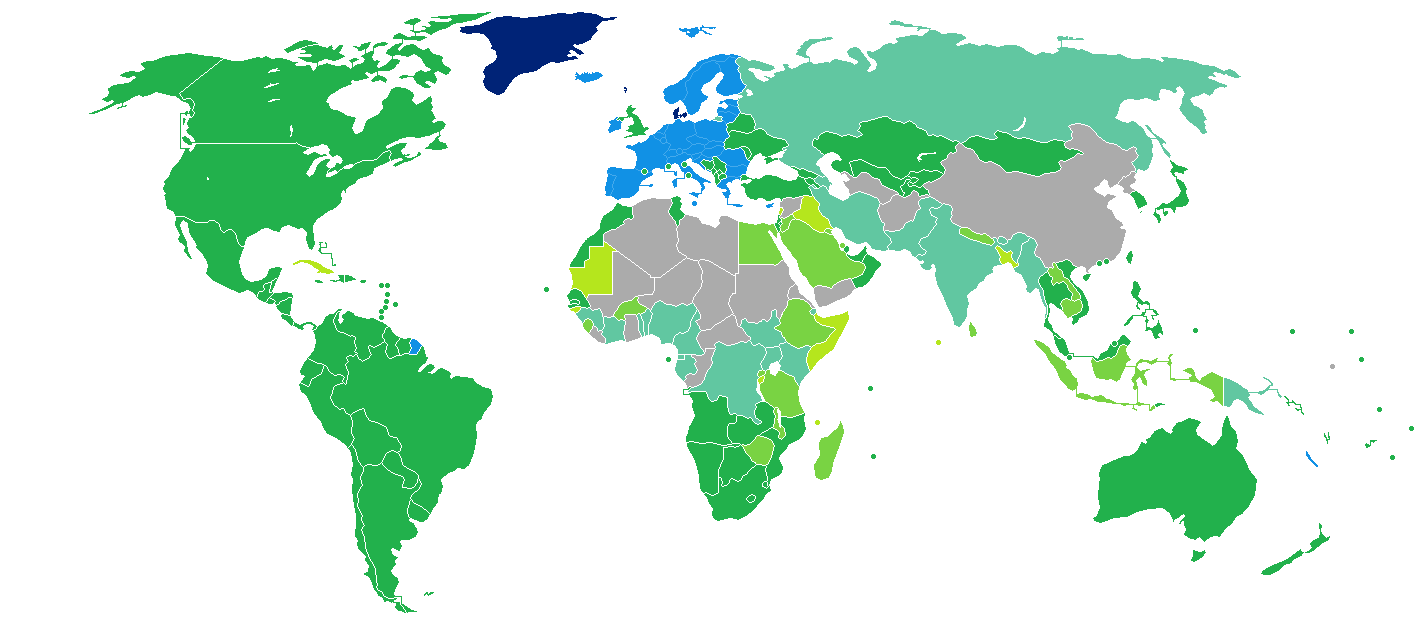This world map displays all continents and countries in a wide array of vibrant colors. To the left, North and South America are depicted in bright, vibrant green hues. In the Gulf and the Caribbean, Cuba and Haiti are rendered in light green. Moving to the right, Greenland is shown in a deep dark blue, while Iceland is illustrated in a lighter blue. Further right, the Nordic countries, including Norway, as well as most of Europe, appear in a light blue shade. However, England and Ireland stand out with a combination of green and blue. Russia is colored mint green, as is most of India. China is shown in gray, in contrast to Mongolia's vibrant green. Africa is depicted using a mix of grays, mint greens, vibrant greens, and lighter lime greens. Australia stands out with a vibrant green, while most of Japan is portrayed in a lighter green. Notably, this map does not include a legend, leaving the meaning of the colors ambiguous.